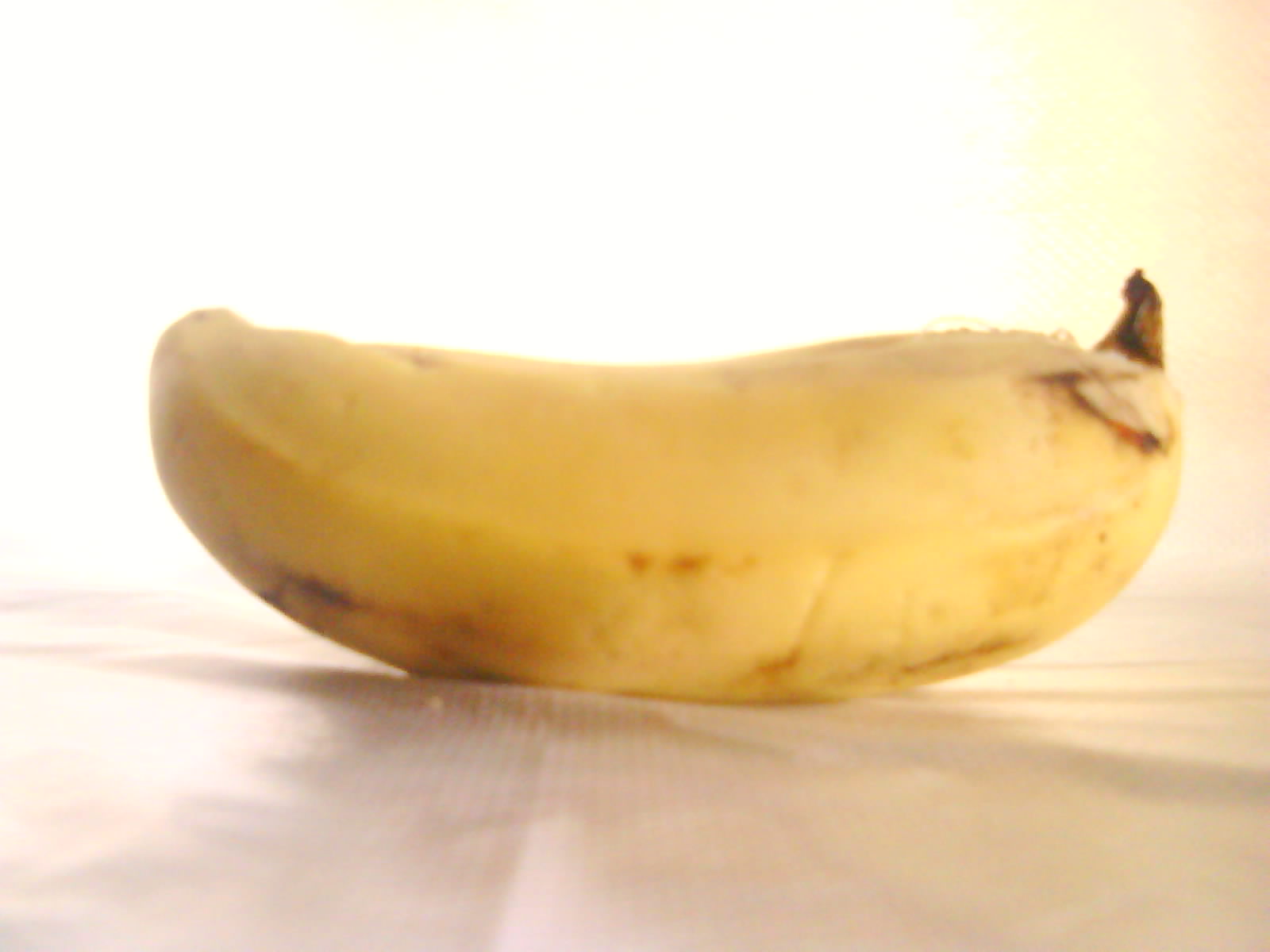A close-up indoor photograph captures an overly ripe banana resting on a white cloth that has a slight wrinkle right below the fruit. The camera is positioned very low, almost at the countertop level, making it difficult to discern the full length of the banana, causing it to appear shorter than it is. The banana is oriented with its stem pointing diagonally up toward the upper right corner, while the other end is slightly tilted up toward the left. The ripe banana is beginning to brown at both ends, near the stem and the bottom. The background is intensely washed out due to a bright light source, which floods in from behind the banana towards the camera, leaving the upper half of the image overexposed and largely whited out. The lower portion of the image reveals some fabric lines and folds that run from the foreground to the background, adding texture to the scene. The image is slightly out of focus, and no text, words, or print are present in the photograph.